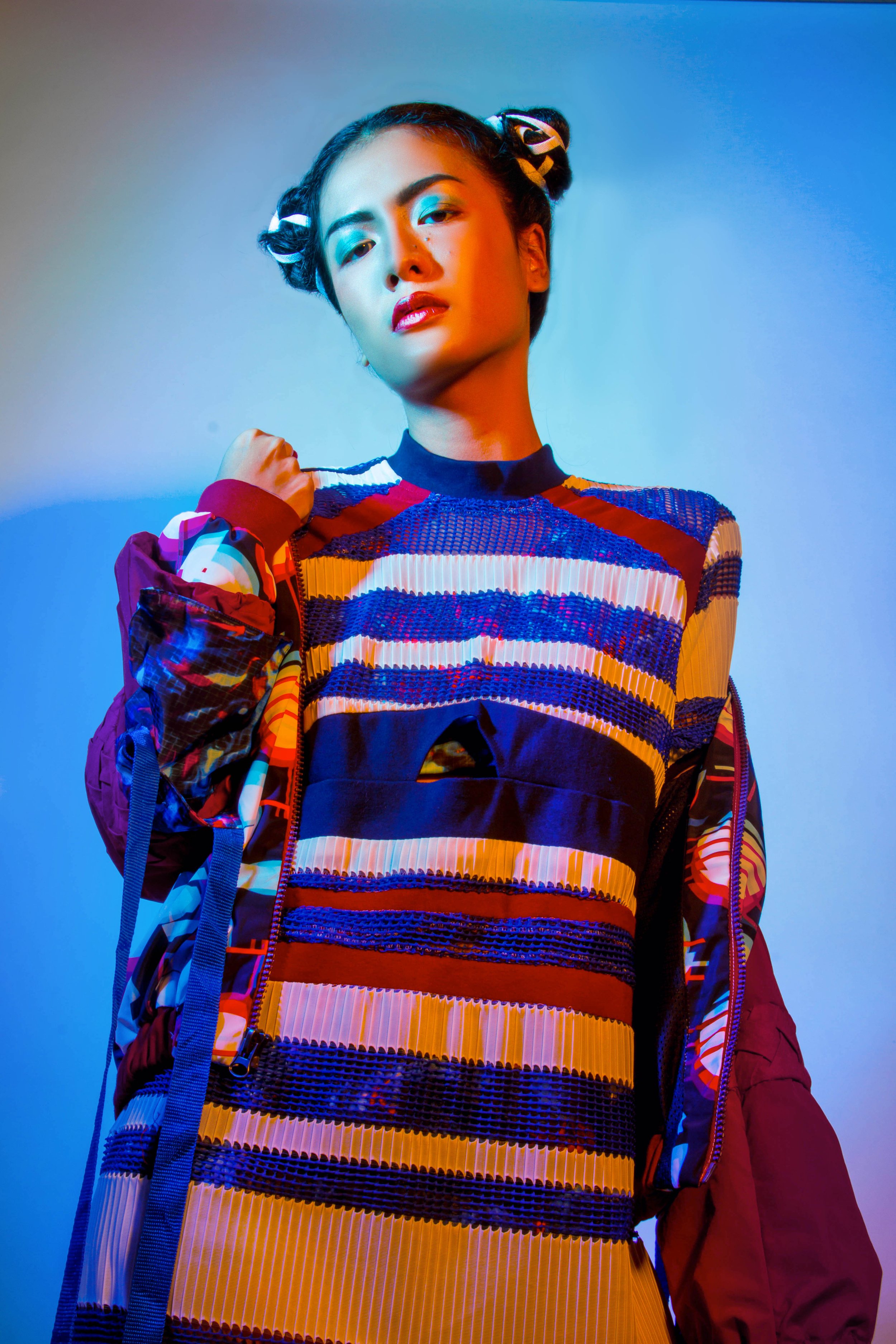The image depicts a young Asian woman with a confident and no-nonsense expression, reminiscent of a model's pose. Her hair is styled in a distinctive manner, parted in the middle and pulled back into high buns on either side of her head, somewhat akin to a Princess Leia style but positioned higher. One of her ears is visible, drawing attention to her symmetrical eyebrows and makeup. She wears a subtle grayish eyeshadow and a moderate red lipstick. 

Her attire consists of a striking blue, red, and white striped dress, which appears to be made of a cozy sweater material, and features baggy sleeves. Draped over her shoulders is a maroon jacket, revealing a colorful inside lining as she appears to be in the process of removing it. She exudes self-assuredness, and her overall look is completed with the suggestion of a bag slung over her right shoulder. The background of the image glows with a light blue hue, adding a vibrant contrast to her poised appearance.